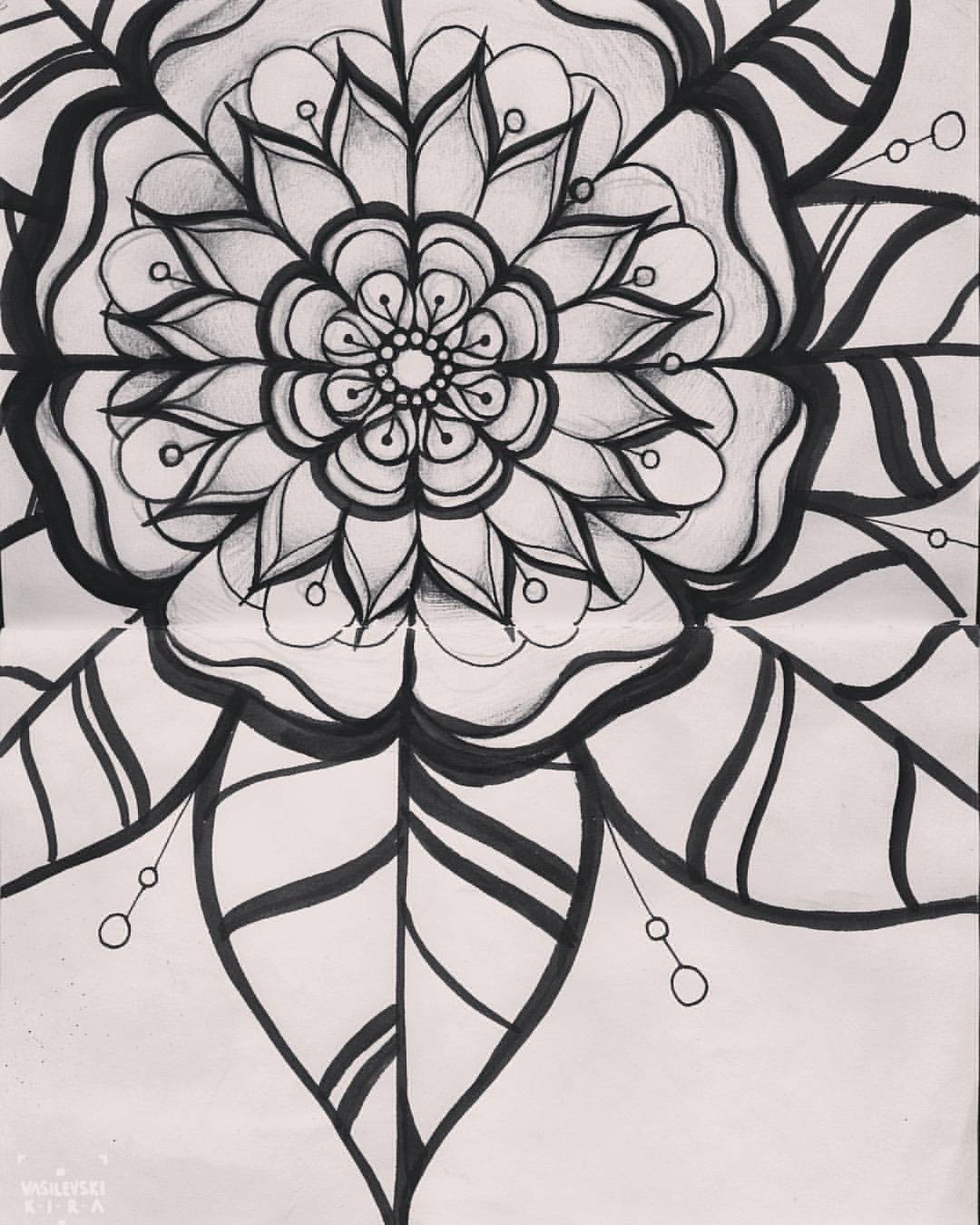This detailed drawing appears to be created with a black marker. In the lower left-hand corner, the names "VASILEVSKI" and "K-I-R-A" are written in white, suggesting the author of the artwork is Kira Vasilevski. The piece prominently features a stylized flower with leaves. The leaves are intricately detailed, showcasing very dark veins that add depth and texture. Some leaves have additional lines adorned with small circles. The flower itself is composed of numerous oval shapes and petals, interspersed with lines and small circles, creating a dynamic pattern. The overall effect is reminiscent of a pinwheel, with varying sizes and intricate details that draw the viewer's eye.